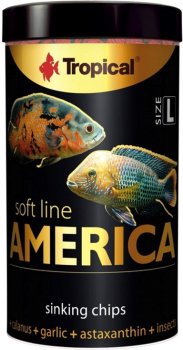This is a high-resolution digital color photograph of a vertically standing bottle of fish food with no surrounding border. The bottle features a sleek black label and a matching black cap. Embellished with gold text, the label prominently displays the word "Tropical" near the top, adjacent to a silhouette of a red fish. Central to the label are two images of fish, aligned vertically and facing opposite directions. Below these images is fine white text stating "Soft Line," followed by "America." Near the bottom of the label, the text "Sinking Chips" is displayed, with a light gold band beneath elucidating the contents of the fish food. Additionally, the top right corner of the label indicates the bottle size with "Size L" along the edge. This meticulously designed bottle stands out due to its sophisticated color scheme and detailed labeling, making it both informative and visually appealing.